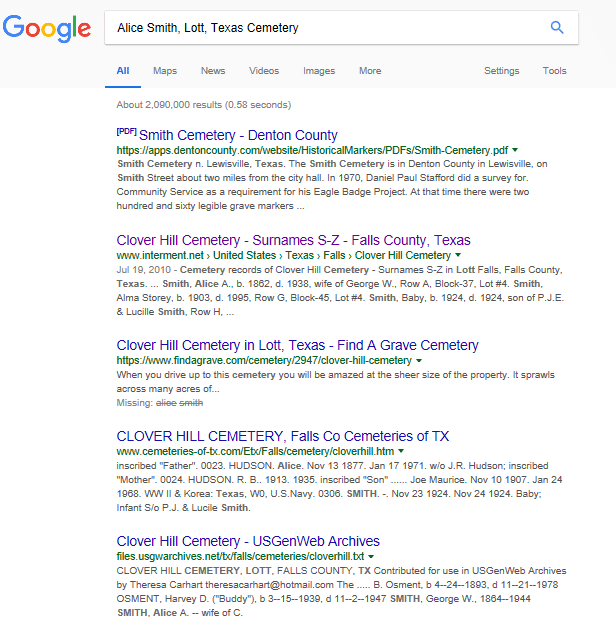The screenshot depicts a Google search results page with the iconic Google logo situated in the upper left corner, adorned in its signature colors of blue, red, yellow, and green. Just to the right of the logo lies the search bar, filled with the query "Alex Smith, lot, Texas Cemetery." Positioned at the far right of the search bar is the recognizable magnifying glass search icon. 

Below the search bar, the navigation tab 'All' is selected and highlighted in blue, indicating the active category. Adjacent to it are other navigation options: Menus, Maps, News, Videos, Images, More, and Settings and Tools.

Beneath the navigation bar, Google displays approximately 2,090,000 results, generated in a swift 0.58 seconds. The search results are displayed in Google's customary format, where the clickable titles are in blue, web addresses in green, and explanatory text in varying shades of gray.

The first search result is for "Smith Cemetery, Denton County," linked to a historic and market-related PDF available on appsdentoncounty.com. The second link, having been previously visited, appears in purple and directs to "Clover Hill Cemetery, Surnames S to Z, Falls County, Texas" on intermittent.net.

Following this, another highlighted search result is for "Clover Hill Cemetery, Lot, Texas" from findagrave.com, showcasing relevant details for Grave Cemetery ID 2947. The subsequent links include cemeteriesoftexas.com, offering information about Clover Hill Cemetery in Falls County, and USGenWebArchives.net, providing access to a Texas cemetery text file related to Clover Hill.

Overall, the user appears to be searching for specific information about a cemetery in Texas, particularly centered on the name Alex Smith and the locality of Clover Hill Cemetery.